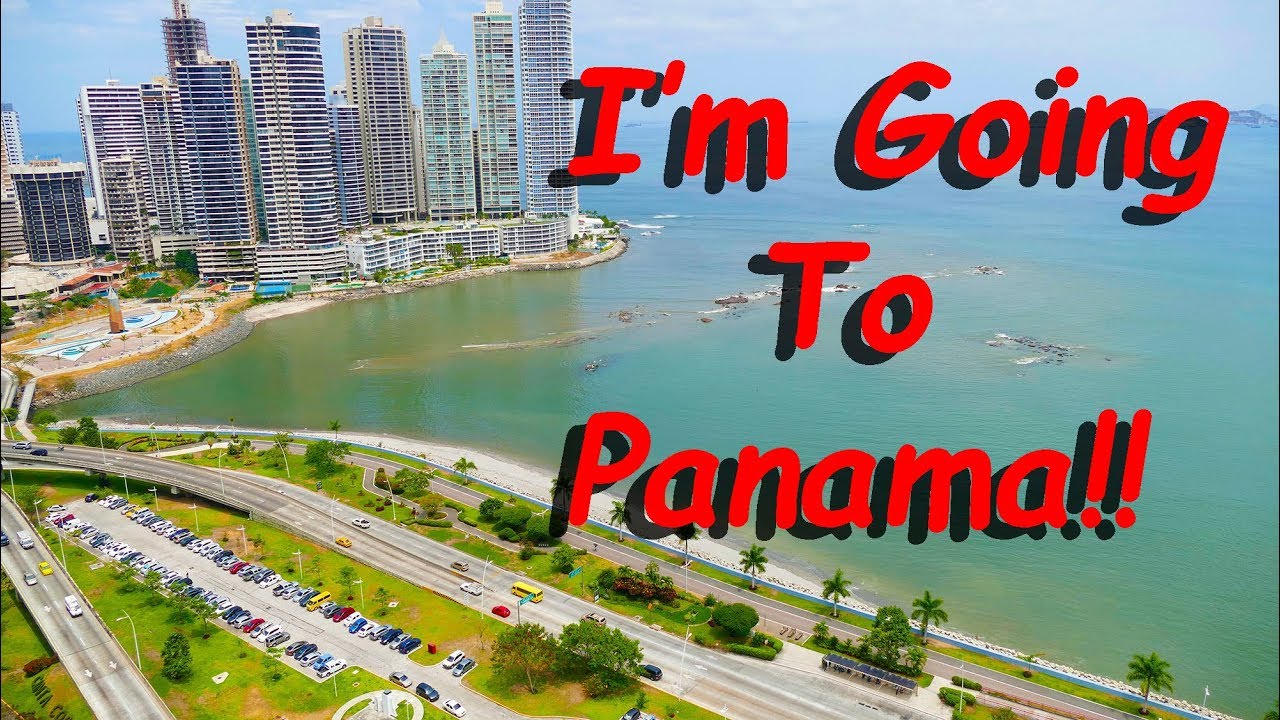The image captures a vibrant coastal cityscape with a bold red and black shadowed text exclaiming, "I'm going to Panama!!" in the foreground. The water is a striking green, contrasting with the clear blue sky above. On the left side, a cluster of tall, gray skyscrapers dominates the scene, indicating a bustling urban area. Below the "P" in "Panama," a stretch of beachfront is visible, lined with evenly spaced palm trees, adding a tropical touch. More traditional trees are scattered inland, interspersed with gray roadways and a sizable parking lot. Elevated ramps lead cars over the land and water, highlighting the city's intricate infrastructure. The overall composition blends urban and natural elements, capturing the dynamic essence of Panama's coastal cityscape.